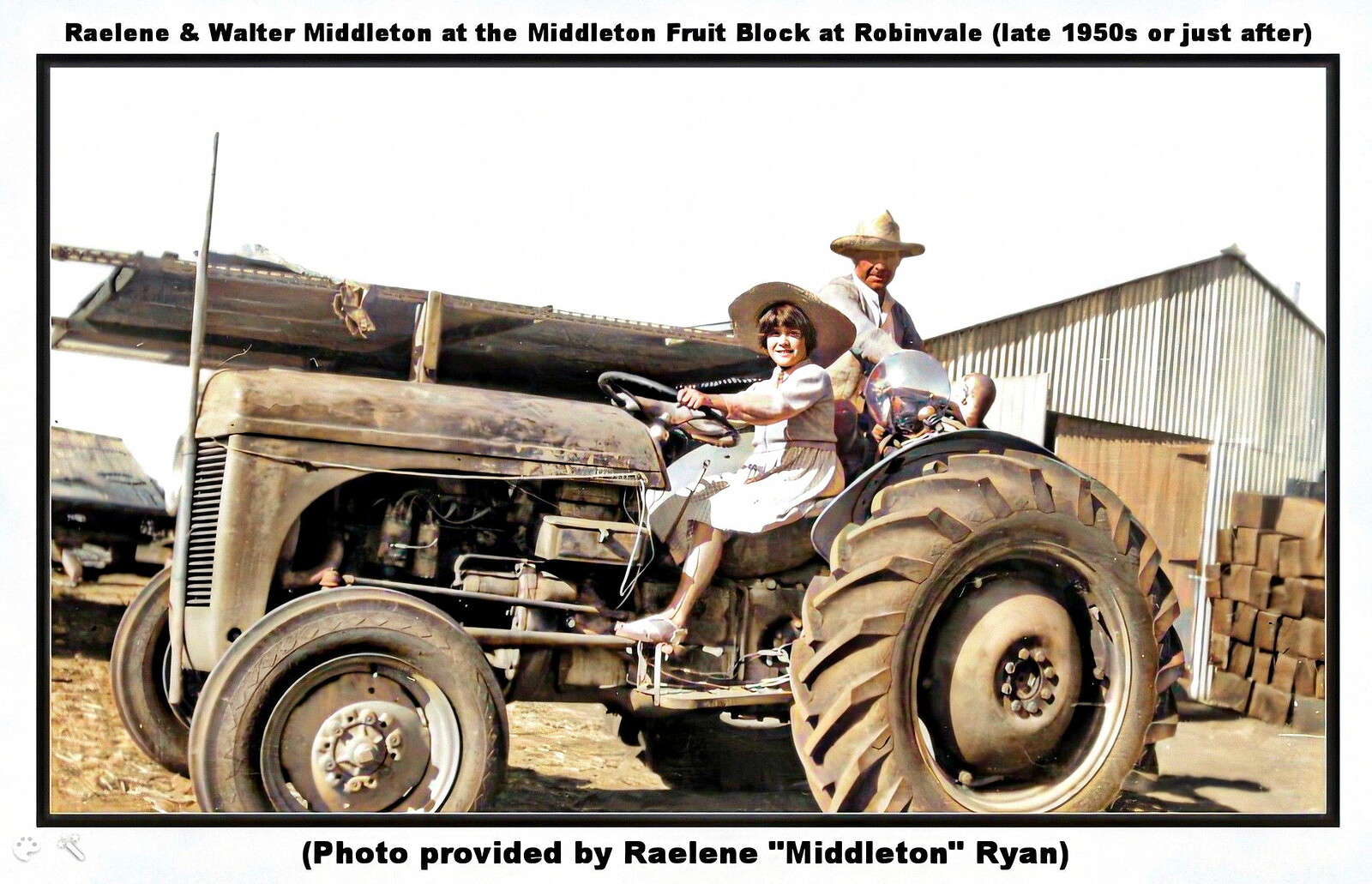In this nostalgic photograph provided by Raylene Middleton Ryan, a young girl is depicted sitting on a large, rusted brown tractor, which appears to have been used countless times. Clad in a dress and a farmer's hat, the girl is seated at the steering wheel, holding it with a firm grip. Behind her, a male figure, likely her father, stands with his arms resting on the tractor, sharing the moment. Both are smiling as they pose for the photograph, looking straight at the camera. The scene is set on a farm, with a dirt road in the foreground. In the background, there is a steel shed or barn, with stacks of boxes or wood piled against its side. The sun shines brightly, casting a warm glow over the entire picture, which has an overall brownish tint. The man is wearing a jacket and also has a hat on. This charming rural scene captures a simple, joyful moment on a bright, sunny day.